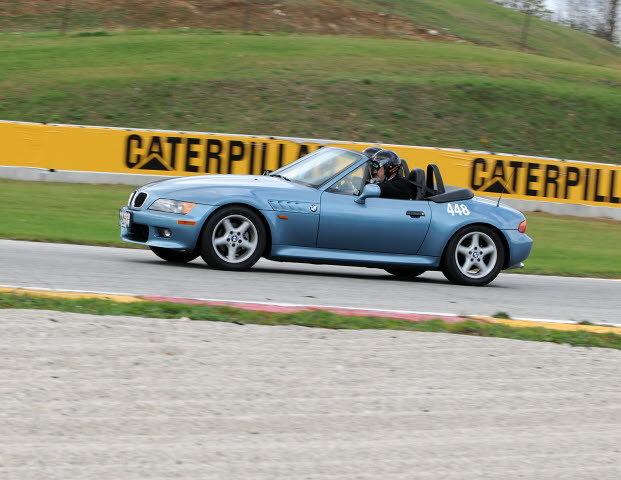The photograph features a small, light blue convertible sports car driving on a grey paved road. The car, viewed from the side, is adorned with the number 448 in white on its rear side panel. Inside the vehicle, the driver, wearing a black helmet, is seated and concentrating on the road ahead. Although not as prominent, a passenger is also visible. The roadway appears to have a small patch of grass growing between two sections of the pavement.

In the background, just behind the car, there is a strip of short, green grass leading up to a yellow boundary wall emblazoned with the word "Caterpillar" in large black letters. Beyond this wall, another stretch of grass-covered ground extends toward an uneven hill. This hill is composed of more green grass and dirt, and a vague, distant fence punctuates its summit. Trees and a clear sky are faintly visible at the top right corner of the image, extending above the crest of the hill, creating a serene backdrop for the dynamic scene.